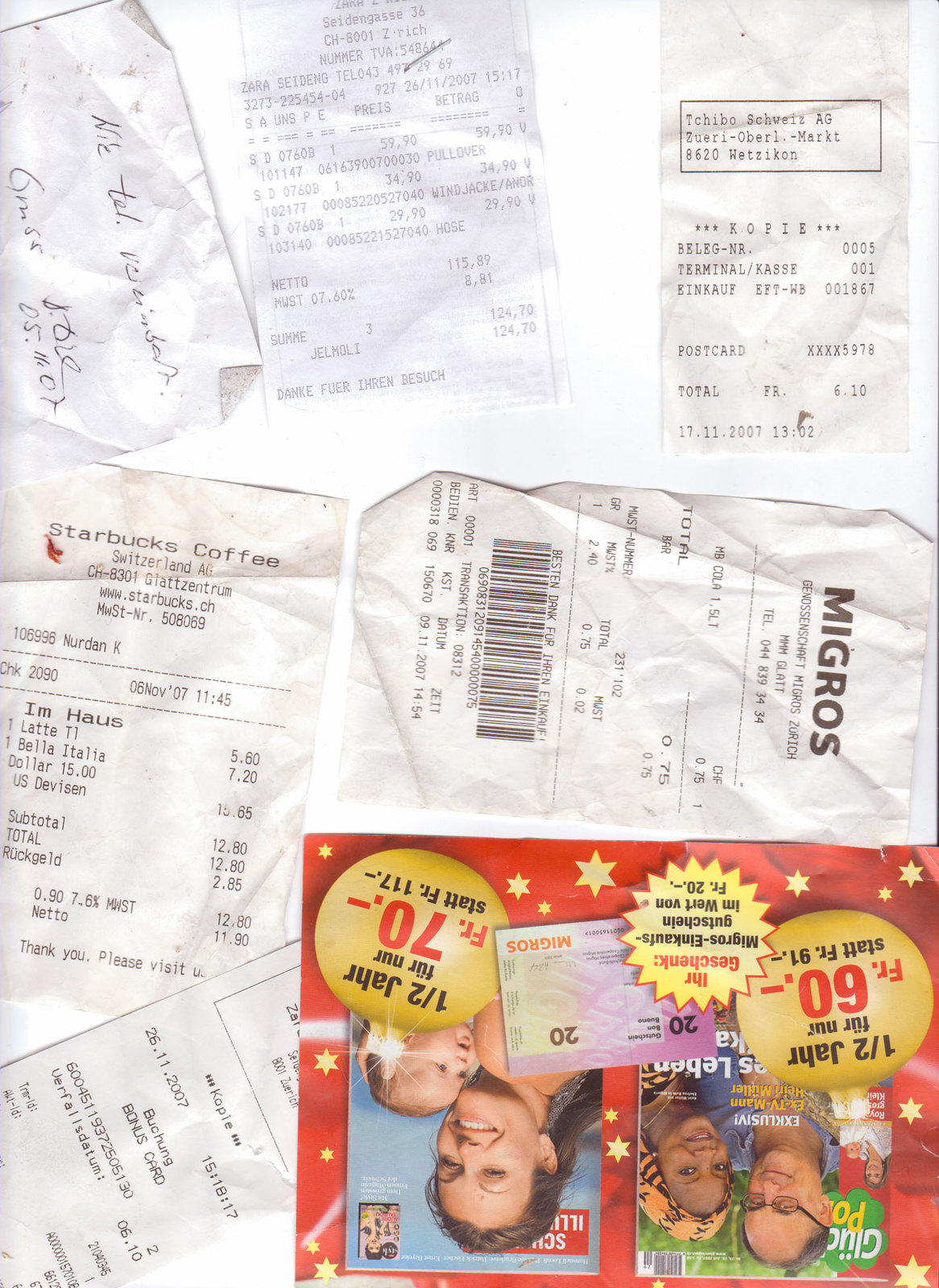The image displays a collection of receipts scattered on a white table. The receipts are from various establishments, including Starbucks and Migros, alongside some that are illegible. Among them, there's an item that resembles a postcard but could also be a receipt or a card. This card, placed upside down, features dual images and includes prices marked as FR.60 and FR.70 in red. Each visible receipt is itemized with specific prices and totals clearly indicated at the bottom. Notably, in the left-hand corner, there is a handwritten receipt adding a personal touch to the assortment. The overall scene presents a diverse array of paper invoices, reflecting a snapshot of assorted transactions.